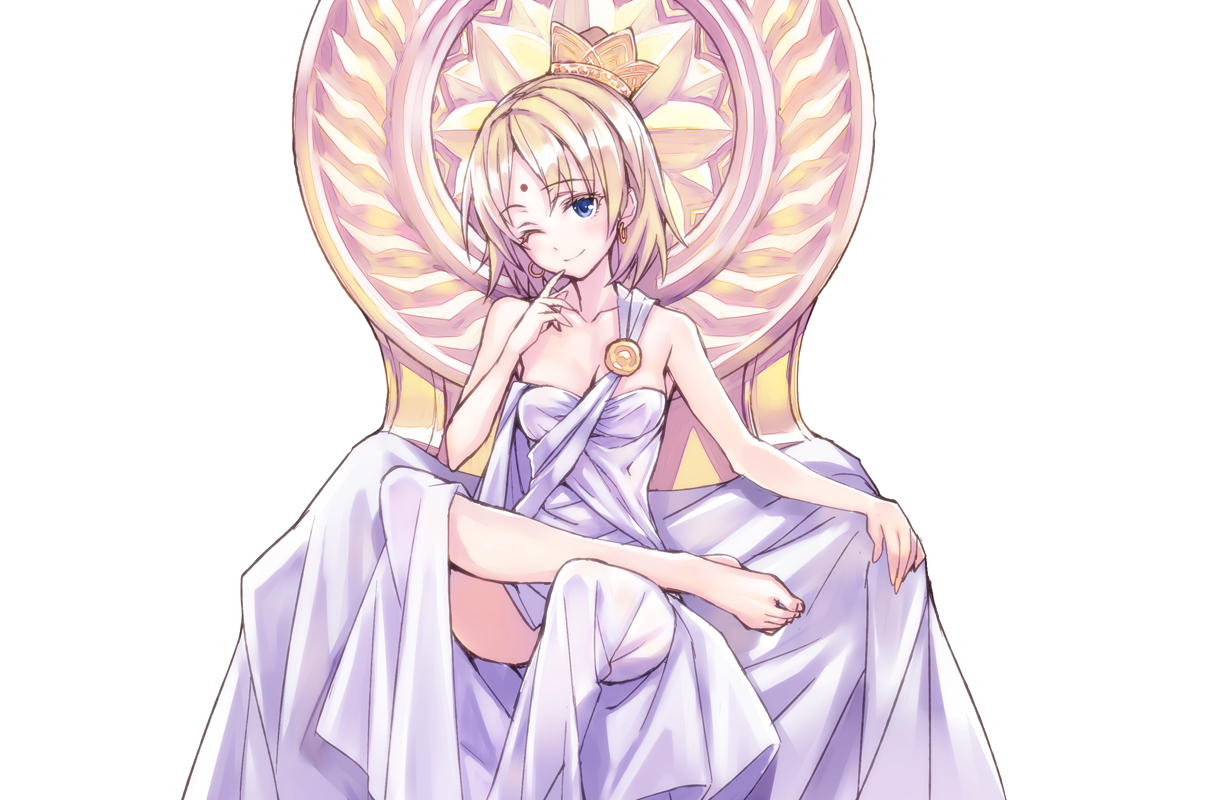The image features a computer-animated, Japanese-influenced anime character, who exudes a regal presence. Dressed in an elegant lavender dress, the character is seated on a luxurious, golden throne. Her blonde hair cascades down, while a crown rests prominently atop her head, further emphasizing her queenly status. Her piercing blue eyes, paired with a distinctive smirk, give her an air of confidence and subtle mischief. Additionally, a unique marking adorns her forehead. The character is posed with one leg crossed over the other, revealing one leg more than the other, adding a somewhat suggestive undertone to her demeanor.